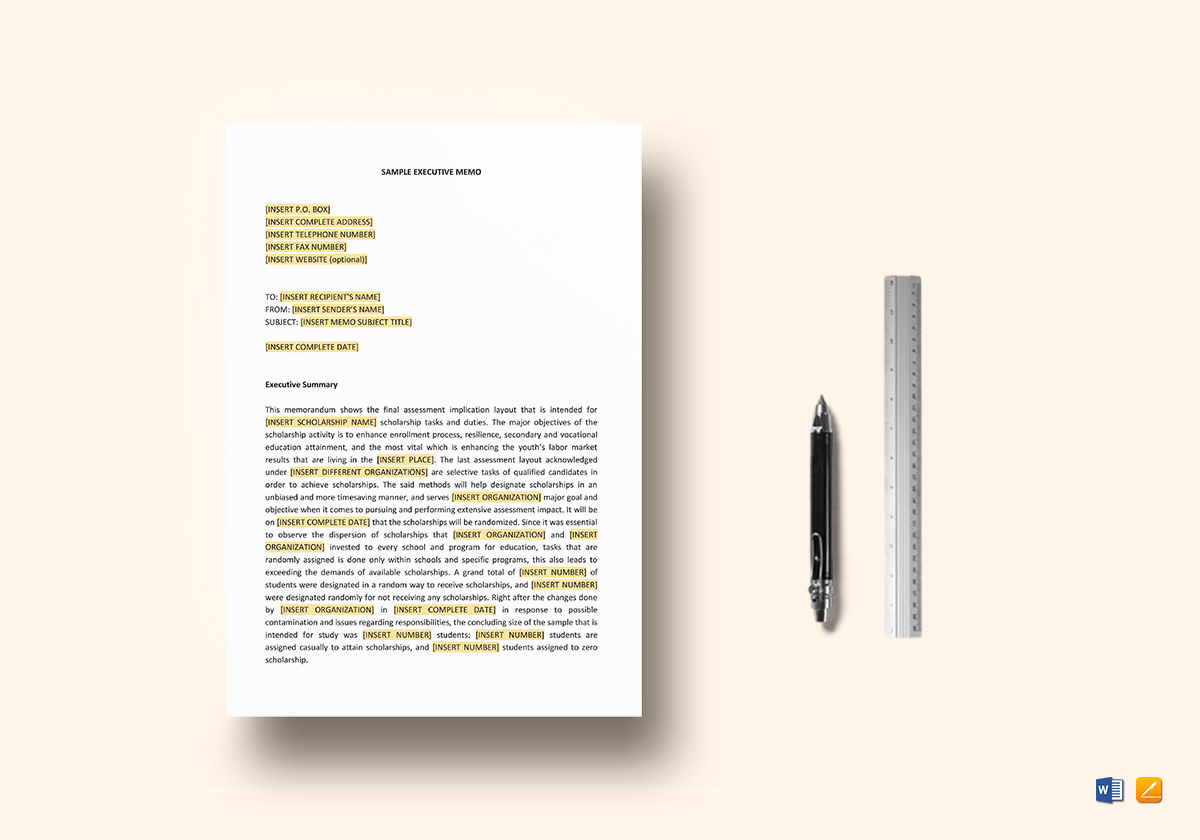The horizontal rectangular image features a pink background with a prominent white piece of paper at its center. The paper appears to be a sample executive memo, marked "Sample Executive Memo" in black writing at the top. The memo includes a section for "Insert P.O. Box," "Insert Complete Address," "Telephone Number," "Fax Number," and "Website Optional," along with fields for "Recipient's Name," "Sender's Name," "Subject," "To," "From," and the "Complete Date." The document is heavily edited with yellow highlighting, drawing attention to the heading, the upper-left paragraph, and some additional text throughout. The letter discusses various attributes of a scholarship program, including its objectives, evaluation methods, and randomized assignment of scholarships.

Alongside the memo on the right side, lies a black and silver ballpoint pen and a silver ruler with black numbering. The ruler is approximately twice the length of the pen. The background, although noted variably, presents as a solid beige color providing a contrasting frame for the memo and the writing instruments. The image offers a detailed view of a professionally formatted document, replete with essential memo elements, annotations, and study-related highlights.